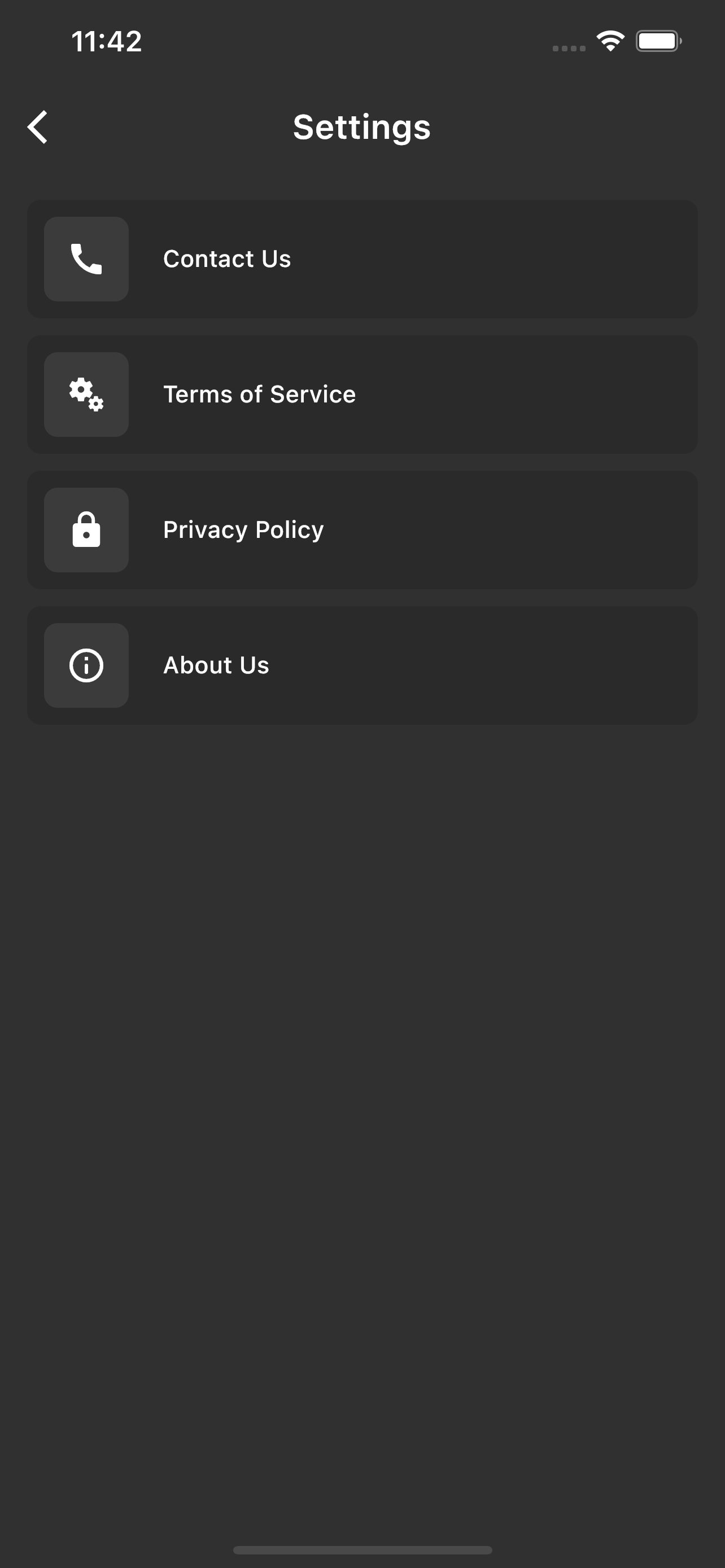The screenshot displays a smartphone interface captured at 11:42 AM, as indicated by the time in the upper left corner. The battery icon in the top right is nearly full, suggesting the device is well-charged. The screen shows the settings page of the smartphone, which is set to night mode or features a dark theme, characterized by a light black background.

In the center top of the screen, the title "Settings" is prominently displayed. Just below it are several menu options, each accompanied by distinct icons:
1. **Contact Us** - Indicated by a phone symbol, suggesting a means to reach customer support.
2. **Terms of Service** - Marked with an icon resembling gears, denoting the legal conditions for using the service.
3. **Privacy Policy** - Represented by a lock icon, indicating information on data protection and privacy handling.
4. **About Us** - Identified by a white circle with an 'i' in the middle, which typically signifies information about the app or company.

Additionally, a back button is located at the top left, allowing users to return to the previous screen. At the bottom, the familiar navigation bar is visible, which can be slid up to return to the home screen. The overall layout is simple and uncluttered, focusing on the essential settings options available to the user.